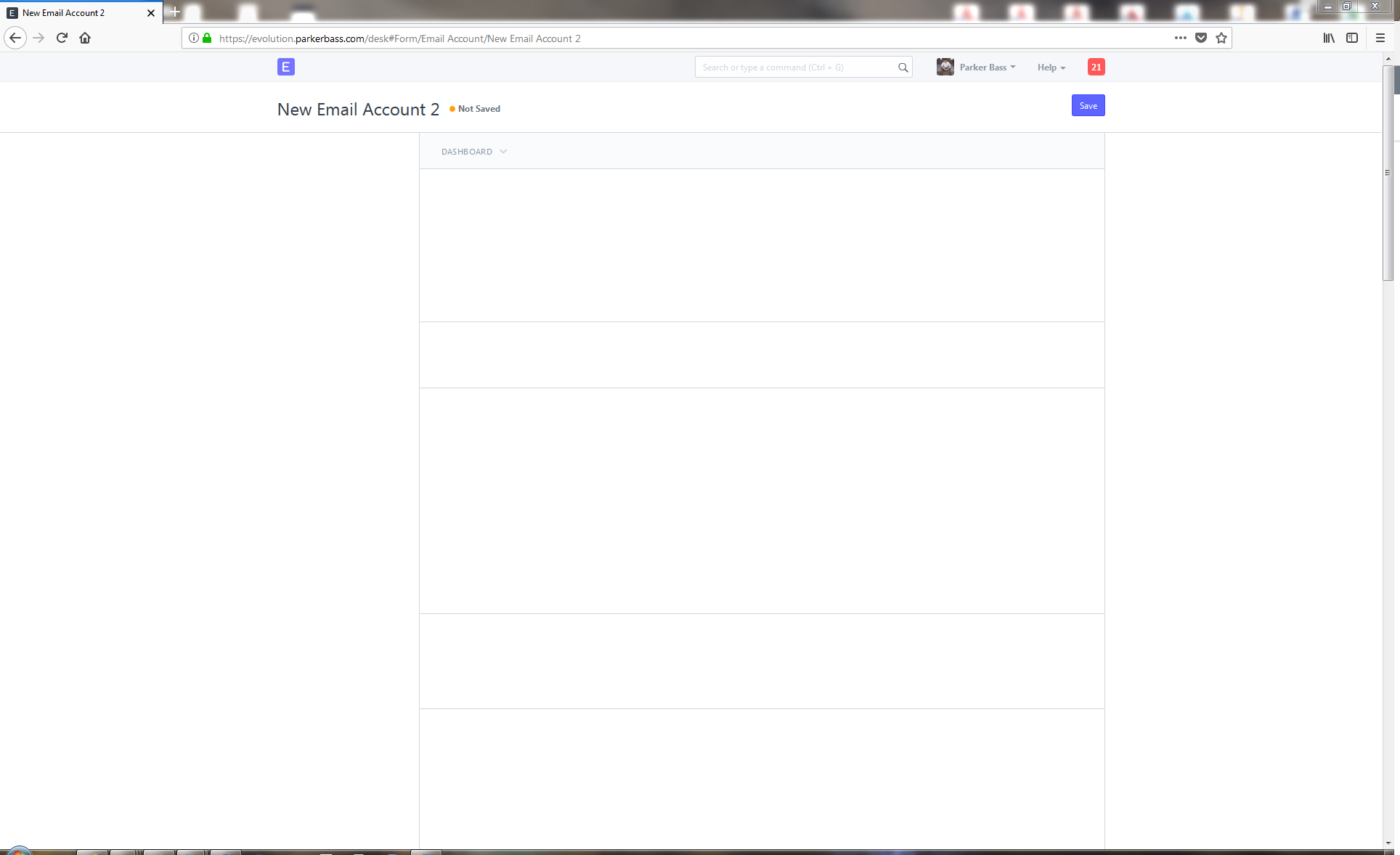The image depicts a screenshot of a computer screen displaying an email interface. In the upper left-hand corner, there is a notification indicating "New email count: 2." Below this, there are several icons: a circular arrow pointing to the left, a gray arrow pointing to the right, a recycle bin, a home button, and an "X" for canceling the current page or tab.

Directly beneath these icons is the URL/search bar, where an HTTP link can be entered. Below this bar, the same "New email count: 2" notification appears once more, accompanied by a status note that reads "Not saved." To the right of this status note is a blue rectangular "Save" button with white text.

Further down the screen, there are three large rectangular input fields intended for typing or entering information. The search bar also features a star icon, allowing users to save the current page as a favorite.